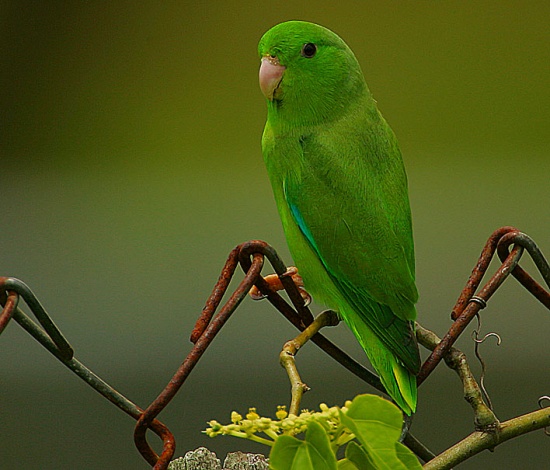This is a photo of a bright green bird perched on top of a rusted brown wire fence, which also features some dark gray areas. The bird, resembling a parakeet or perhaps a young parrot, showcases an enchanting shade of kelly green mixed with lime green. It sits upright with its wings folded, facing slightly to the left. The bird has small, black eyes and an orange-ish brown beak and claws. Wrapped around the fence are some winding vines with a few leaves, creating a touch of natural greenery in the scene. The background is a beautifully blurred gradient of spring green, with a darker patch in the upper left corner, emphasizing the vibrant colors and details of the bird in the foreground.